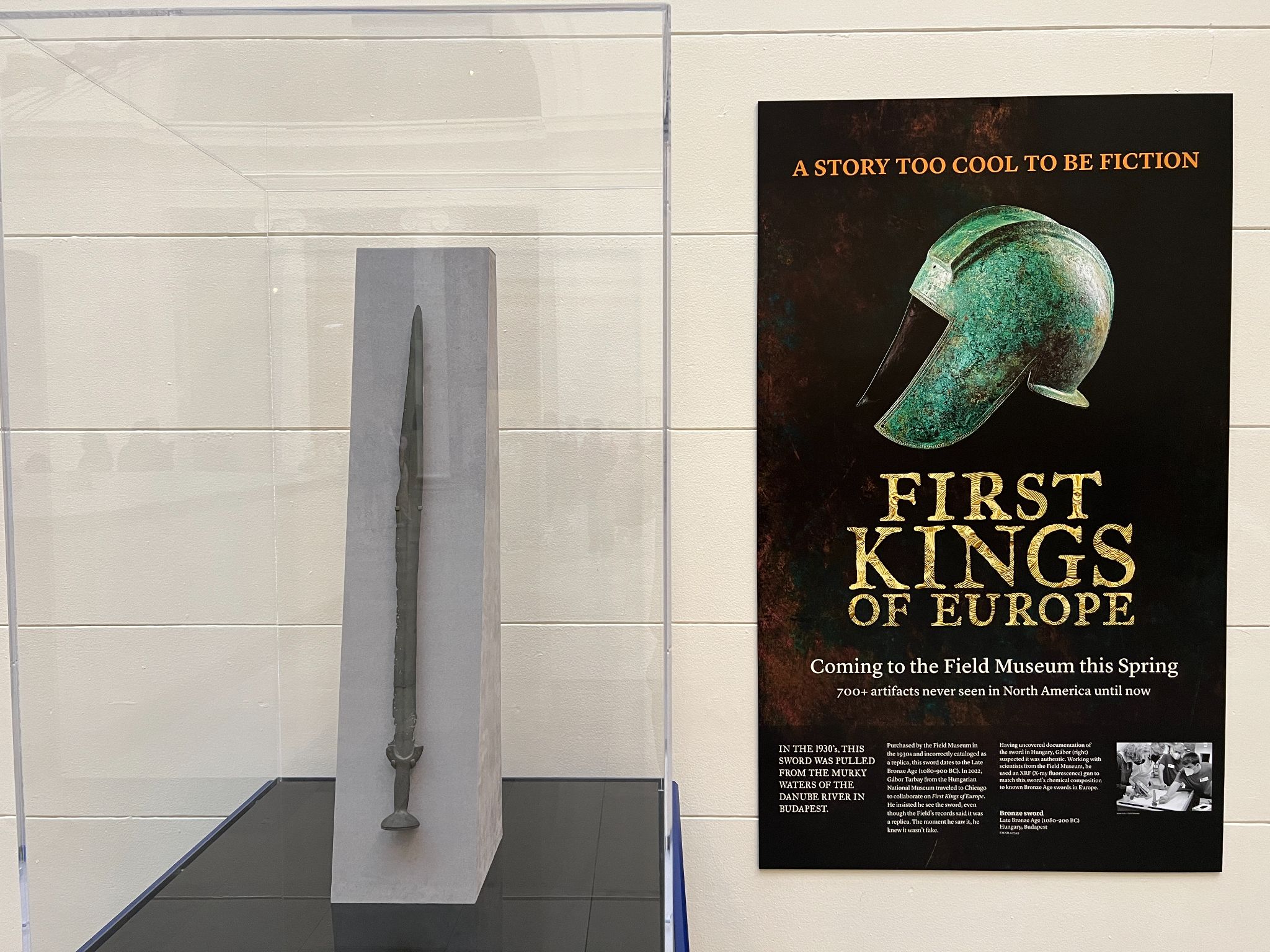The photograph depicts a museum exhibit with an off-white background. On the left side of the image, a long, dark-colored sword, likely made of stone, is mounted vertically on a gray block that sits atop a black table, enclosed in a glass case. The wall on the right side features a poster with prominent orange capital letters at the top, stating, "A STORY TOO COOL TO BE FICTION." Below this, a green helmet is displayed, facing left. In much larger gold capital letters, the text reads, "FIRST KINGS OF EUROPE," followed by white capital letters announcing, "COMING TO THE FIELD MUSEUM THIS SPRING." Additional text, including "700+ artifacts never seen in North America until now," and historical details about the sword being pulled from the Danube River in Budapest in the 1930s, is also present but difficult to read due to its small size. The colors in the image include white, green, black, blue, brown, and orange, creating a detailed and inviting preview of the upcoming exhibit.